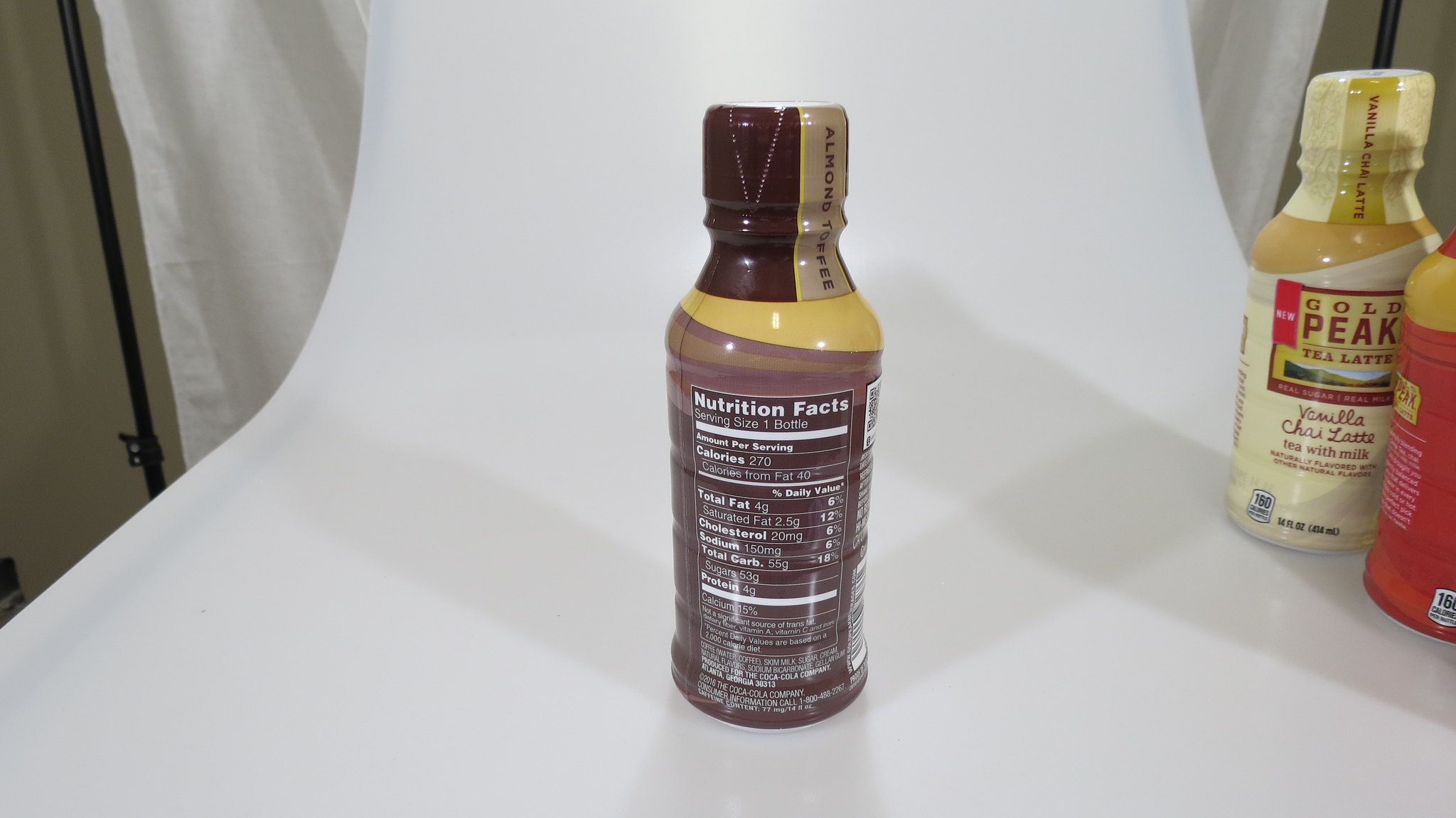The image depicts three beverage bottles arranged with varying levels of prominence. In the foreground, a bottle features a label denoting "Vanilla Tri-Latte" under the brand Gold Peak. The label is designed with a yellow square and carries text indicating it's a tea latte mixed with milk. The label's intricate details include nutrition facts, showcasing 47 calories and breakdowns of total fat, cholesterol, sodium, and total carbohydrates. The reflective surface of this bottle captures light, creating an interesting visual effect.

Adjacent to this, on the right, stands another bottle with a red label, adorned with yellow at the top. It casts noticeable shadows, adding depth to the composition. 

In the background, partially visible, is a third bottle. The visible side of this bottle suggests a minimalistic design, hinting at sequences of white fabric and gray metal poles that frame the scene. The upper part of one bottle appears wrapped in plastic with dotted lines forming a triangle shape, indicating it’s peelable. The entire arrangement suggests an atmosphere of a casual yet meticulously organized display with a dream-like focus on the central bottle. The varying colors and textures—from the white and brown lines on the nutrition facts to the shadows—make for a compelling and detailed visual presentation.